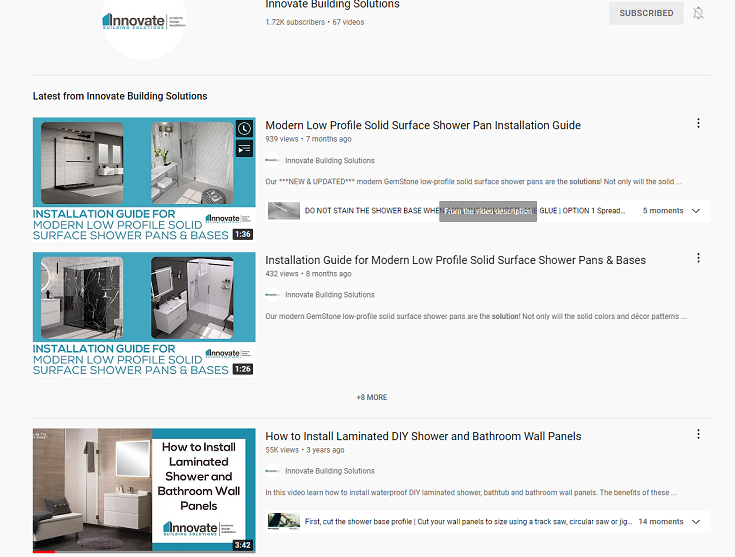The image showcases the homepage of the Innovate Building Solutions website. Prominently displayed in the center is the website's name. In the top left corner, there's a small Innovate Building Solutions logo, while the top right features a subscribe button and a notifications bell icon.

Just below the top navigation bar, a series of images on the left display various modern solutions the company offers. These include a step-by-step installation guide for a contemporary low-profile solid surface shower pan and base. The visuals depict sleek, futuristic sinks and showers, which are likely video thumbnails, given the timestamps such as "1:26" and "3:42" displayed on them.

To the right of these images, there are corresponding titles and view counts for each item. For example, the first video has been viewed 939 times as of 7 months ago, the second one has 432 views, and the third one—clearly very popular—has amassed 55,000 views over the past 3 years. This section succinctly provides users with insightful information about the company’s innovative offerings and their reception over time.